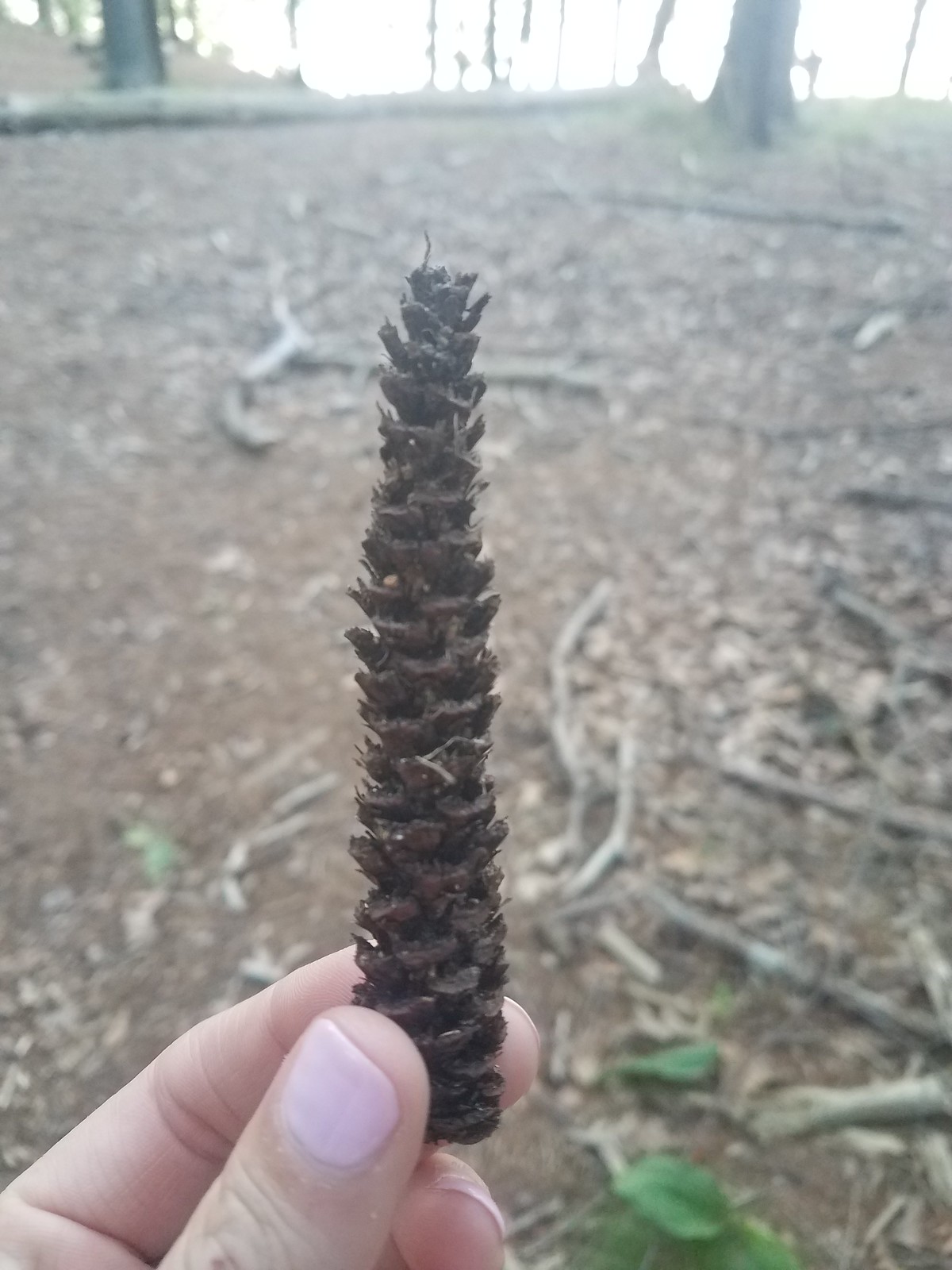In this image, a female with freshly painted pink nails is holding a slender, elongated brown pine cone between her thumb and index finger, positioned towards the bottom left-hand corner of the frame. The pine cone, though narrow and small in diameter, stands out due to its tall, Christmas tree-like appearance, and is held up clearly in focus against a blurred backdrop of a forested area. The forest scene includes scattered sticks, leaves, and shadowy tree trunks. A log lying horizontally stretches from the left towards the center-right, nestled among the ground debris. The background remains softly lit with diffuse daylight illuminating the scene. The hand and pine cone dominate the image, with the intricate, scaly structure of the pine cone contrasting sharply against the natural, yet indistinct forest environment.